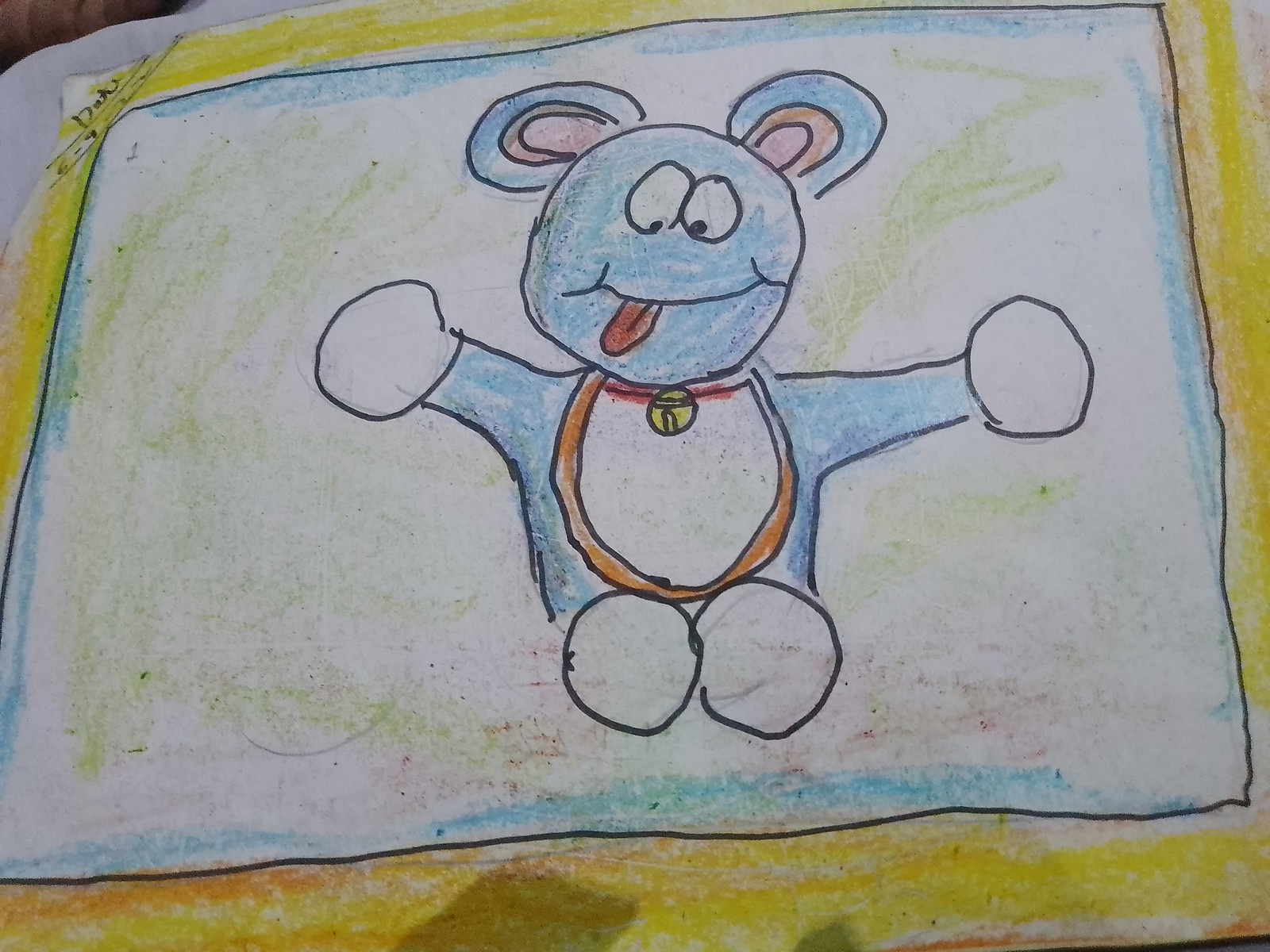In this detailed color photograph, we see what appears to be a child or an artist's whimsical drawing prominently featured at the center. The drawing occupies nearly the entire frame of the photograph, with a portion cut off at the upper right corner. The illustration is bordered by a yellow edge, likely created with crayon or colored pencils, providing a bright frame around the central figure.

Dominating the center of the drawing is a simple, cartoonish rendition of a bunny rabbit. This light blue bunny, possibly a depiction of a stuffed animal, is seated upright, mimicking a human posture. It extends its two front paws forward, adding to its anthropomorphic charm. The bunny's face captures a playful, fun-loving expression with a goofy smile. One corner of its mouth is playfully tilted, revealing a tiny tongue. Its eyes are simplistic yet endearing - two small circles placed closely together with dotted pupils.

Complementing its whimsical facial features, the bunny has long ears drawn with minimalistic strokes. These ears are predominantly blue, accented with a touch of pink on the inside, enhancing the bunny's endearing and approachable appearance. The combination of vibrant colors and naive artistry gives the drawing an innocent, joyful feel, perfectly capturing the essence of carefree creativity.